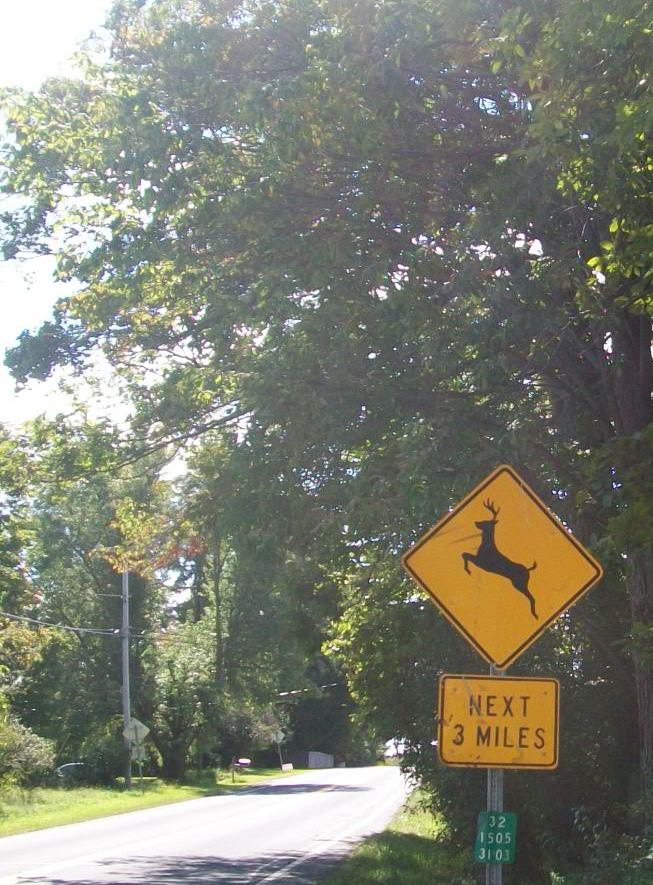The photograph captures a roadside scene dominated by a large tree that encroaches over the road, providing a natural frame for the composition. Starting from the bottom left corner, the road winds its way into the background, eventually disappearing behind the tree. In the foreground, prominently positioned in front of this tree, stands a multi-layered signpost. The topmost sign is diamond-shaped, featuring a black silhouette of a leaping deer against a yellow backdrop, indicative of a wildlife crossing zone. Below this, a rectangular sign with black text on a yellow background cautions, "Next 3 Miles," suggesting that drivers should remain alert for deer over this distance. The lowest sign on the post is a utility marker, displaying the numbers "32-1505-3103" in white text over a green background.

Opposite the signpost, across the road, a utility pole punctuates the scene, with at least two wires stretching into and out of it, serving as a reminder of human infrastructure in this otherwise natural setting. The back of another diamond-shaped sign is visible on this side, hinting at additional road safety advisories. Further off in the distance, a mailbox stands on the roadside, adding a touch of rural charm. Dominating much of the photograph is the expansive tree, whose branches spread out and hang over the road, casting dappled shadows on the pavement and creating a serene, picturesque atmosphere.